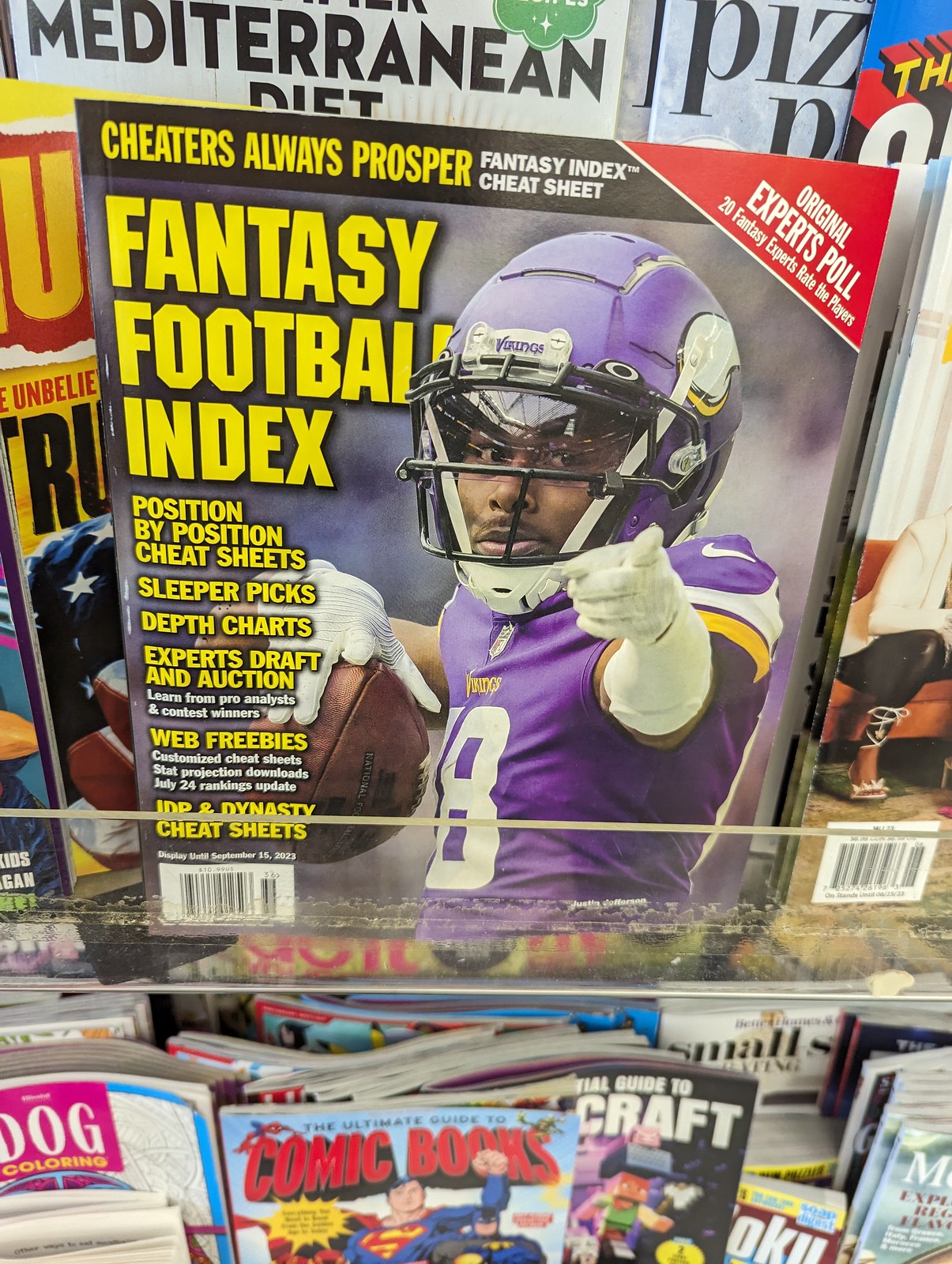This image showcases a plastic display stand in a store, filled with an array of magazines and books. The central focus is a magazine titled "Fantasy Football Index," prominently featuring Minnesota Vikings player Justin Jefferson on the cover. He is depicted in his purple uniform, number 18, pointing with his left hand while holding a brown football with his white-gloved right hand. The magazine cover includes bold yellow text stating "Cheaters Always Prosper" and offers various features like position-by-position cheat sheets, sleeper picks, depth charts, expert drafts, auctions, and web freebies. Surrounding this magazine are other publications, including a Mediterranean diet guide, a comic book with Superman on the cover, a dog coloring book, an official Minecraft guide, and a magazine showing a woman sitting on a brown couch. Visible barcodes can also be seen on some of these items.